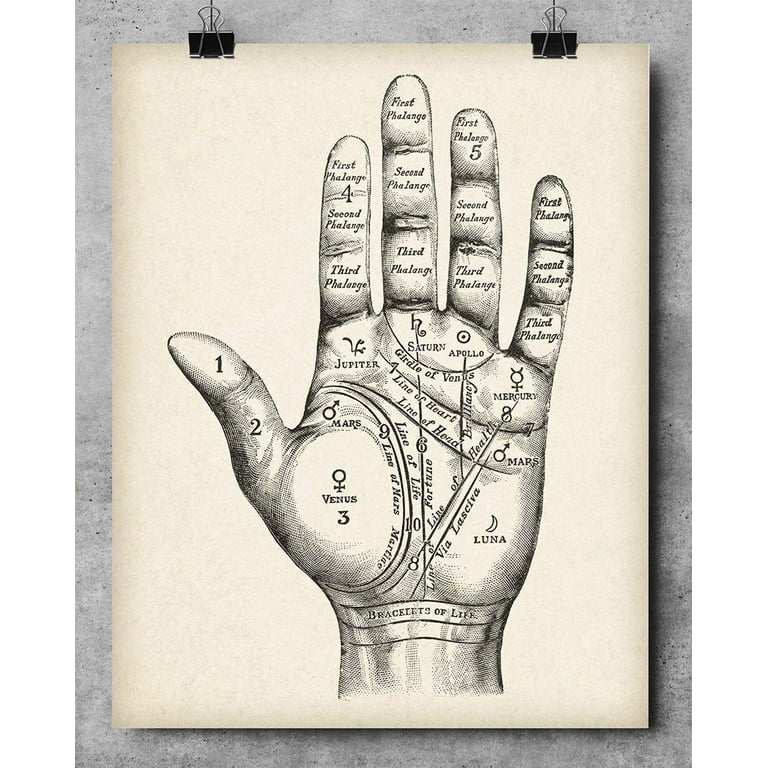The photograph features a vertical rectangle with a gray, cement-like background. In the center, there is an off-white, yellowing piece of paper held up by two black clips at the top corners. The paper displays a detailed, black-and-white sketch of a left hand, palm up, surrounded by numerous labels. Each section of the hand is intricately marked, indicative of palm reading practices. The fingers, divided into three sections called flanges, are annotated with numbers: the thumb is labeled one, with its base as number two, the pointer finger as four, and the ring finger as five. The palm areas are named with terms such as Venus, Jupiter, Saturn, Apollo, and Luna, and significant lines like the line of heart, line of life, and bracelets of life are also highlighted. The thorough labeling extends to various features, correlating different regions with specific meanings in line with the belief system portrayed.